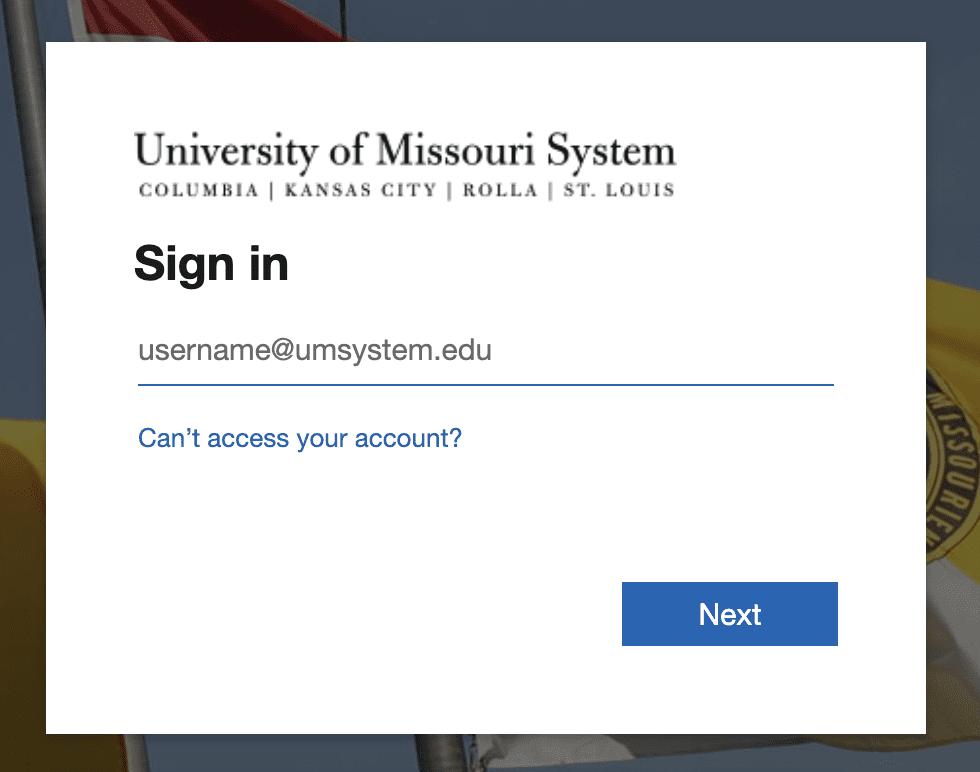The image appears to depict a login page for the University of Missouri System. At the top of the page, there is a yellow flag icon and a grey pole. Below this, a prominent white square captures attention. The page identifies itself as belonging to the University of Missouri System, encompassing the campuses of Columbia, Kansas City, St. Louis, and Rolla. The login section features black bullet points and prompts users to sign in with their username, specifically formatted as username@system.edu. There is also a link provided for users who cannot access their accounts, stating "Can't access your account?". Finally, a blue rectangle button with the word "Next" is situated on the right side for progressing through the login process. The edges of the page are grey at the top left, completing the clean and organized layout.